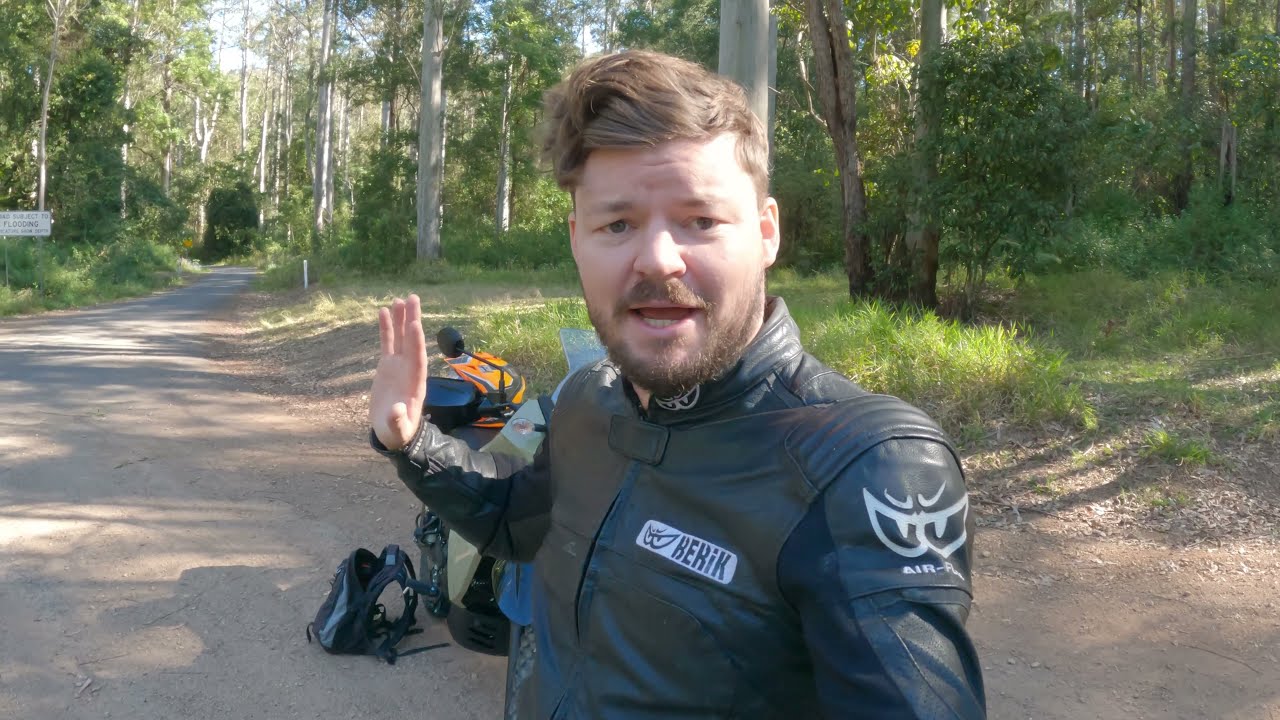A highly detailed photograph captures a young man standing on a narrow, dirt country road flanked by trees. His light brown hair has a wavy, swooped style, complemented by a light brown beard and mustache. He is dressed in a black leather motorcycle jacket bearing a distinctive logo labeled 'K'E'K'K' or possibly 'H-E-H-I-K,' alongside a decal of angry eyes, mirrored on his left shoulder patch. His gray eyes add intensity to his expression as he raises his right hand in what appears to be mid-gesticulation, perhaps explaining something or recording a vlog. 

In the background, an orange motorcycle stands with a yellow helmet perched on its seat, alongside an open backpack lying on the ground. The scene is set against a backdrop of looming trees and a road sign warning of potential flooding. This scenic, yet solitary landscape emphasizes the sense of adventure and exploration, indicative of someone documenting their journey through the woods.